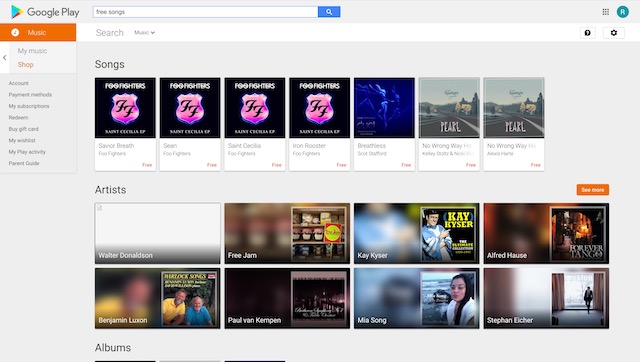This image captures a low-resolution, reduced-size screenshot of a Google Play Music interface. At the top of the interface, the Google Play icon is prominently displayed, featuring the recognizable triangular symbol adorned in Google's signature colors. Adjacent to the icon is a search bar marked by a magnifying glass icon, with the placeholder text reading "free songs." On the upper right-hand side, there's a grid icon composed of nine small squares, situated next to the user's initial, "R."

Beneath these navigation elements, a gear icon for settings and a question mark for help are also visible. The primary section of the screen showcases a series of free songs listed horizontally. Each entry displays an album cover, including those from the Foo Fighters and a band named Pearl, with a "Free" label in the bottom right corner of each song's box.

Below the songs section lies the "Artists" menu, presenting various artists in larger horizontal rectangles. The mentioned artists range from Kay Kaiser and Alfred House to Mia Song, Pearl, and Paul Van Kempen, although the text appears slightly blurry.

The screenshot cuts off just as it reaches the "Albums" section, hinting at a continuation if one were to scroll further. On the left side of the interface, a vertical menu offers options such as Account, Payment Methods, Subscription, Redeem, Buy Gift Cards, My Wishlist, My Play Activity, and Parent Guide. These options allow users to manage their purchases and account details. The background of the interface is a subtle, soft pale gray, providing a neutral backdrop for the various elements displayed.